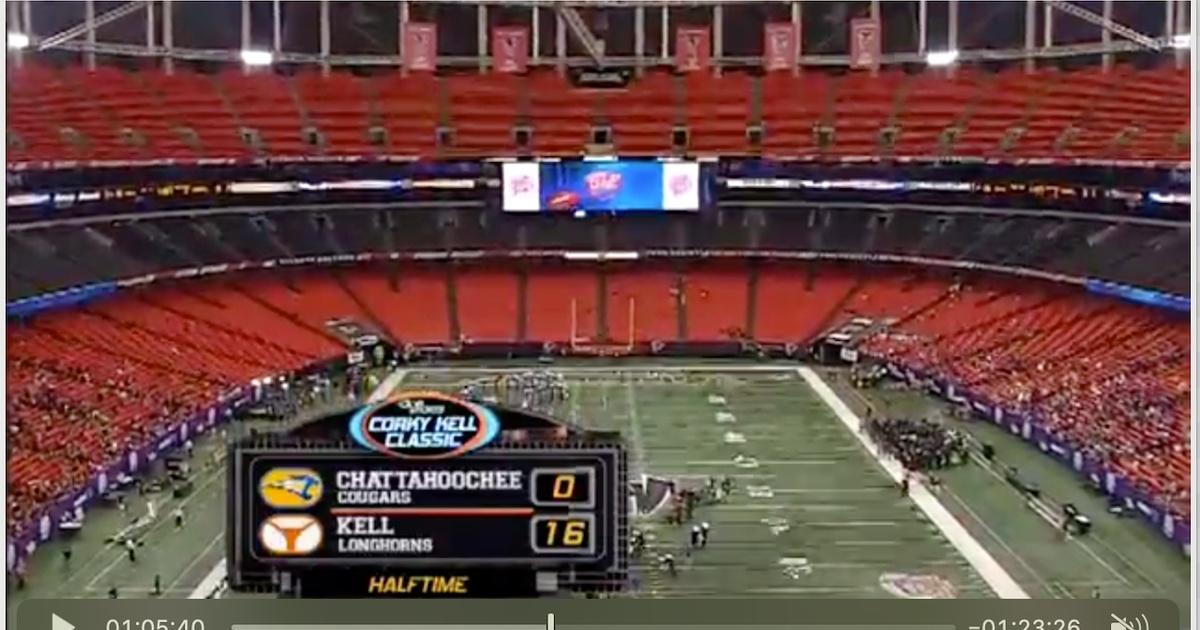The image depicts a screenshot from a video stream of an American football game, specifically during the Corky Kell Classic. The scene is an aerial view of a large stadium, captured from an elevated position approximately 100 feet above the ground. The stadium appears sparsely populated, with only about 10% to 20% of the seats occupied, primarily on the left and right sides, while the upper seating ahead is mostly empty. A large television scoreboard is visible, displaying the score: Chattahoochee Cougars, 0, and Kell Longhorns, 16. It is currently halftime. Additionally, the video player interface at the bottom of the screen, possibly from an iPhone, shows the viewer is one hour, five minutes, and 40 seconds into the video, with one hour, 23 minutes, and 26 seconds remaining.